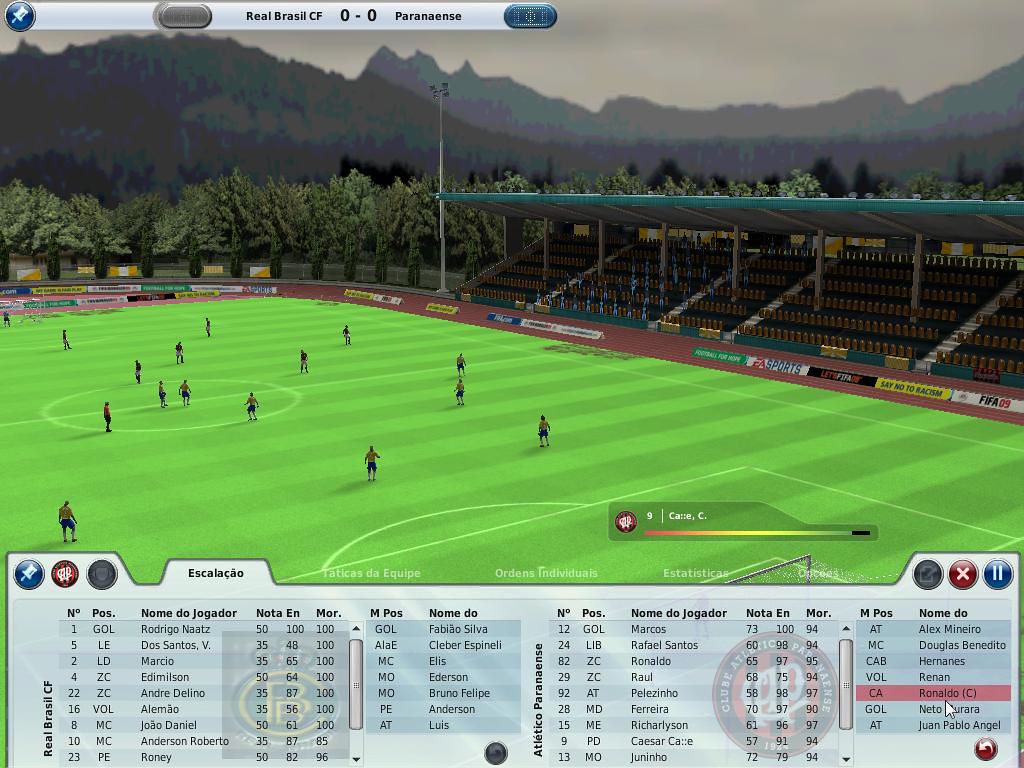The image depicts a soccer video game scene set within an expansive, lush green field. The viewpoint is from a zoomed-out camera perspective, capturing the full scope of the field and making the players appear quite small. On the right side of the field, stands are filled with spectators, distinguishable by their red and blue attire, although they remain fairly indistinct due to the distance. Supporting an overhead structure, green-colored pillars are also visible. In the background, a picturesque setting includes an array of trees and distant mountains under a grayish sky.

The game's user interface (UI) is prominent, providing key details about the match. In the top left corner, a scoreboard displays "Real Brazil CF 0-0 Parananes," indicating the current score of the game. At the bottom of the screen, a detailed UI panel shows a list of player names along with various statistics, scripted in what appears to be Spanish. This UI element is large and contains numerous details critical for gameplay, immersing the player further into the virtual soccer experience.